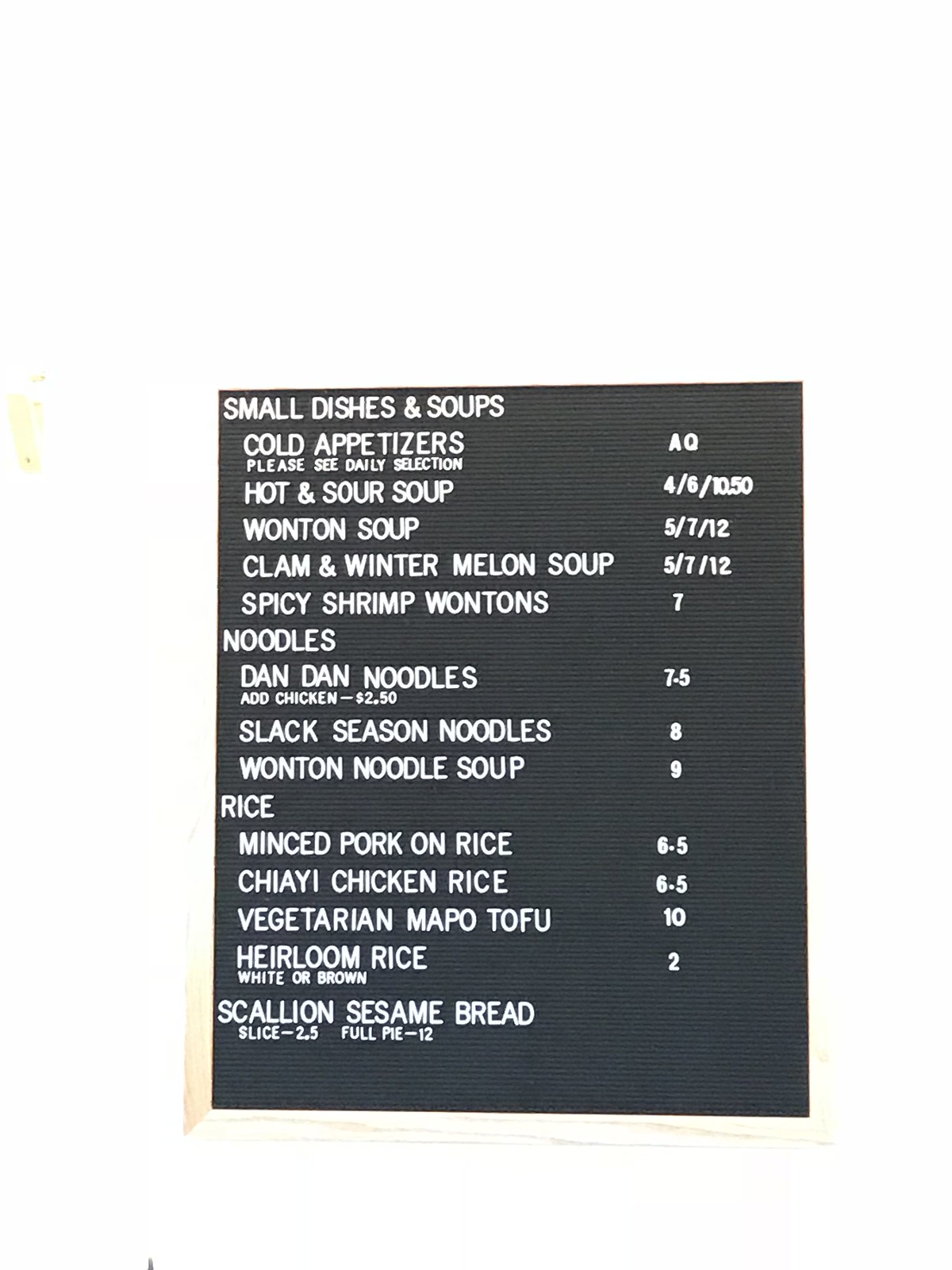The menu, set against a black background, details a variety of dishes, neatly categorized under small dishes and soups, reminiscent of classic diner platforms. At the top, it notes "Cold Appetizers" with a request to "Please see the daily selection."

Following this are the soups:
- **Hot and Sour Soup:** Offered in three sizes: $4, $6, and $10.50
- **Wonton Soup:** Available for $5, $7, and $12
- **Clam and Winter Melon Soup:** Priced at $5, $7, and $12

Next, the noodle dishes are listed:
- **Spicy Shrimp Wonton Noodles:** $7
- **Dan Dan Noodles:** Priced at $7 per serving; you can add chicken for an extra $2.50
- **Slack Season Noodles:** $8
- **Wonton Noodle Soup:** $9

From the rice section, you have:
- **Minced Pork on Rice:** $6.50
- **Chicken Rice:** $6.50

Vegetarian options include:
- **Vegetarian Mapo Tofu:** $10

There's also an heirloom rice option available in white or brown, accompanied by "Scallion Sesame" slices priced at $2.50 each. Additionally, a "Full Pie" is available for $12.

This menu layout offers an organized selection of both classic and unique dishes.